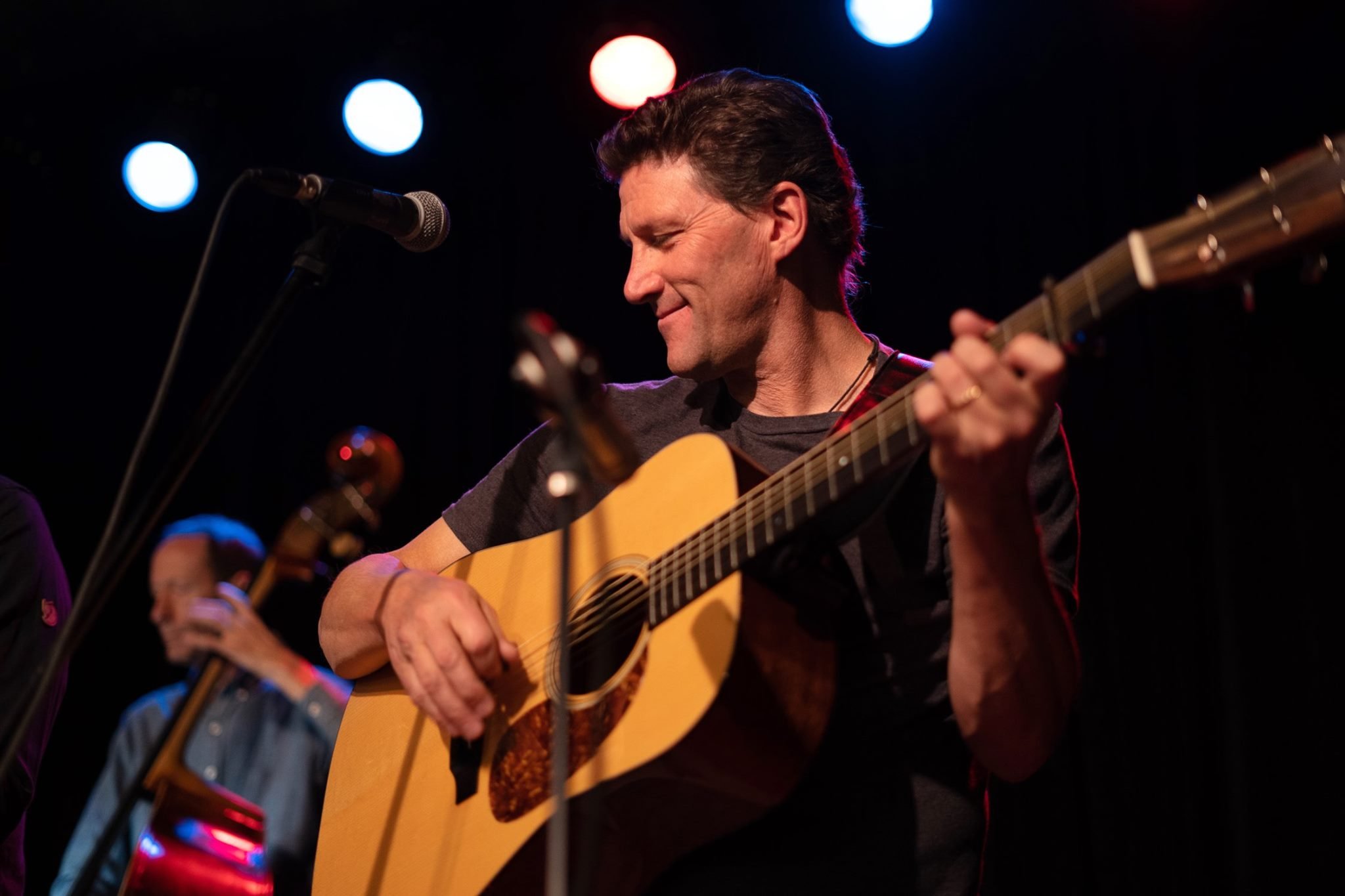In this landscape-oriented photograph, predominantly set against a dark background, the focal point is a middle-aged Caucasian man with short brown curly hair, centered within the image. He is depicted smiling and holding an acoustic guitar with a yellowish-tan front, strumming it gently with his right hand. He is dressed in a dark gray or brown t-shirt, and a ring is visible on one of his fingers. Positioned directly in front of him is a microphone on a stand, while another microphone stand is to his left. 

In the bottom left corner, slightly behind the main performer and over his right shoulder, the top half of another man, wearing a blue button-up shirt, is visible. This man is playing a larger, reddish stand-up bass. The scene is illuminated by three round white lights shining down from the top left corner towards the center, reinforcing the sense that this is a live musical performance. The detailed arrangement and coloration of the setting, including shades of tan, brown, gray, light blue, white, and black, contribute to the atmospheric and engaging depiction of the concert scene.